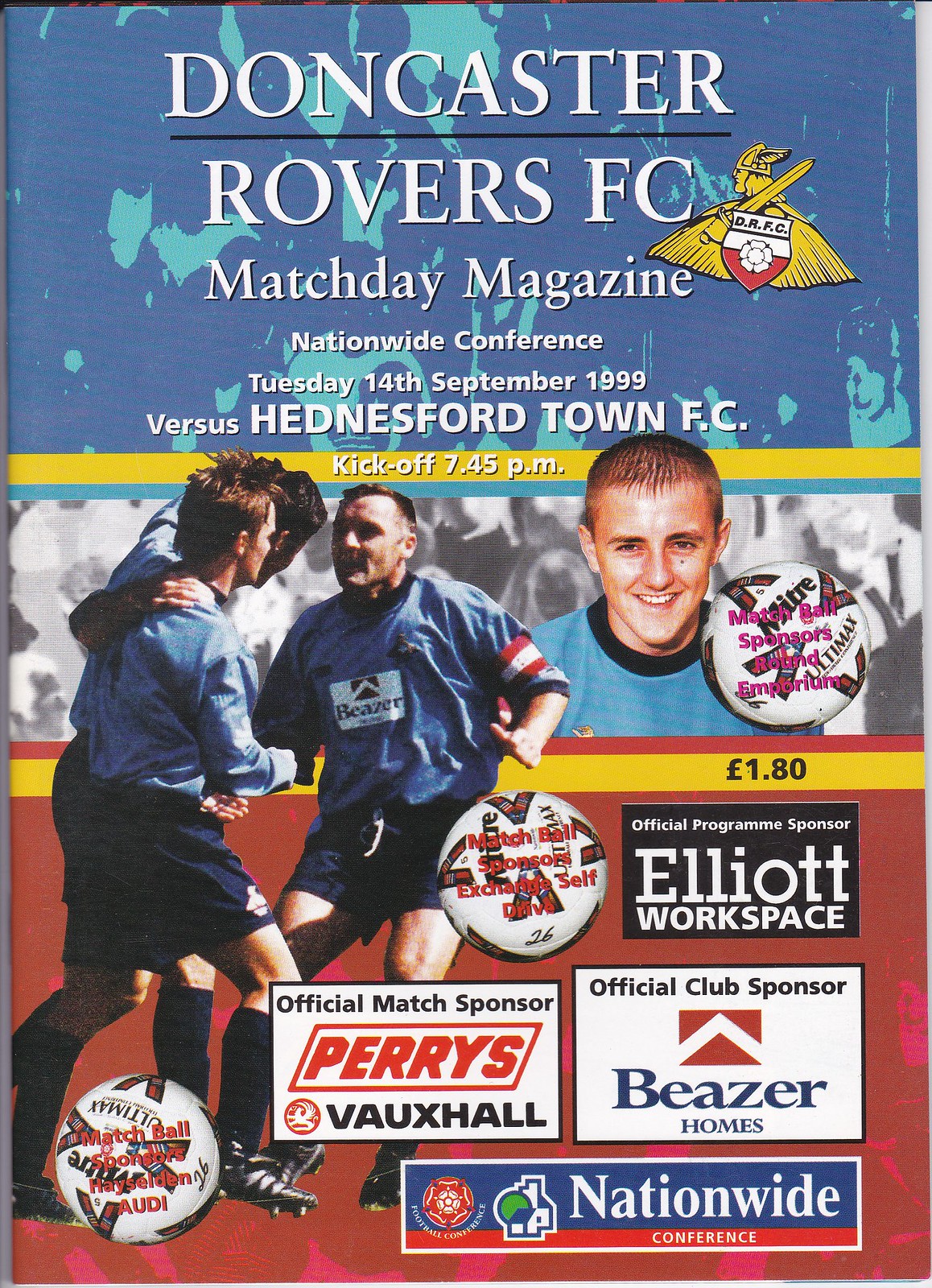The image depicts the cover of a match day program for Doncaster Rovers FC, prominently showcasing the event on Tuesday, 14th September 1999, against Hednesford Town FC, with a kickoff at 7:45 PM. At the top, in white text, the title "Doncaster Rovers FC" is displayed next to a golden Viking insignia holding a sword. Below this, in smaller white text, it reads "Match Day Magazine, Nationwide Conference." The central part of the cover features a large photograph of three football players clad in powder blue jerseys and dark blue shorts, seemingly celebrating a goal, with an additional headshot of a smiling player to the right. Surrounding these images are multiple footballs, each branded with different sponsor names like "Round M," "Exchange Self-Drive," and "Hazelden Audi." The design is stylized with a blue and light green background on the top half and a reddish backdrop on the bottom half, giving the cover a dynamic and vibrant appearance. Sponsors' logos are positioned at the bottom.